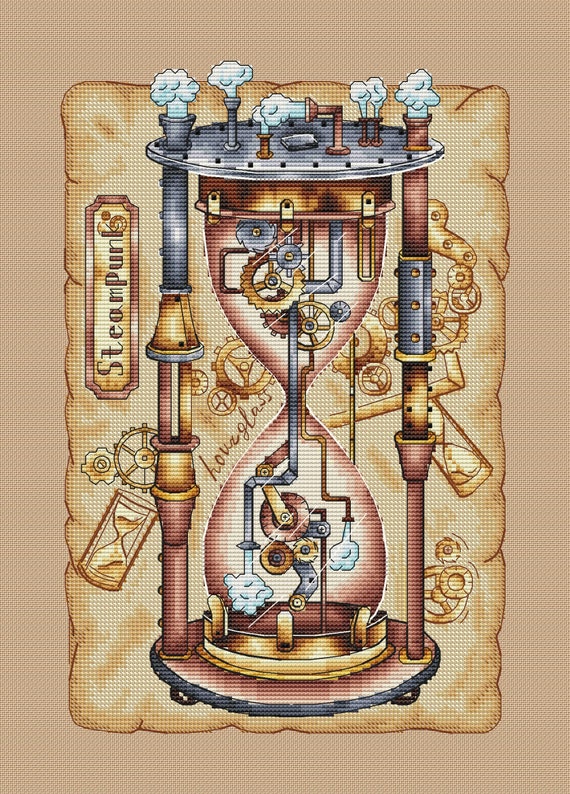The image showcases a digitally designed, stylistic rendering of a steampunk-themed hourglass. The background features a tan to peach-like color resembling aged, torn paper, bordered by a darker brown, giving it an antique and vintage appearance. The centerpiece, an hourglass, displays an intricate array of gears and tubes in bronze, gold, and silver shades instead of traditional sand. The hourglass is crowned with metal pipes emitting steam, adding to its mechanical and robotic essence. On the left side of the hourglass, the word "Steampunk" is vertically inscribed, clearly indicating the theme. The overall design cleverly mimics the texture of needlepoint or embroidery, enhancing its artistic and woven tapestry appearance.